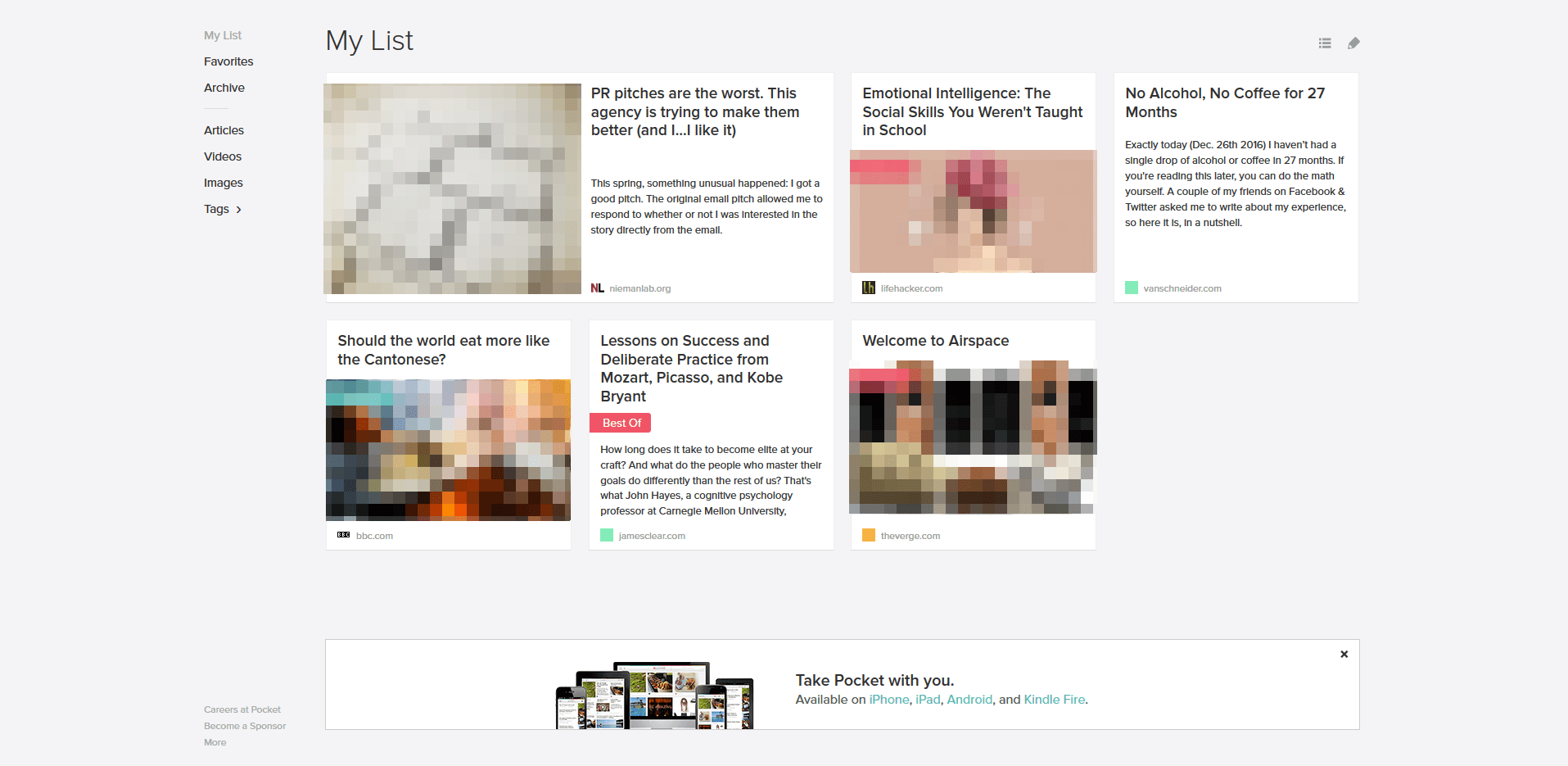This image, captured from a website's screen under the section titled "My List," showcases a grid layout with a top row of four squares and a bottom row of three squares. Each square contains either a picture or accompanying information. 

The first square in the top row features a blurry, pixelated image. Beside it, the text reads, "PR pitches are the worst, this agency is trying to make them better, and I like it." The description continues: "This spring, something unusual happened—I received a good pitch. The original email pitch allowed me to respond to whether or not I was interested in the story directly from the email."

The second square in the top row next to the first contains text that says, "Emotional Intelligence: The Social Skills You Weren't Taught in School," paired with another pixelated image, suggesting a privacy preference.

In the third square, the text reads, "No Alcohol, No Coffee for 27 Months." It details, "As of today, December 26, 2016, I haven't had a single drop of alcohol or coffee in 27 months. If you're reading this later, you can do the math yourself. A couple of my friends on Facebook and Twitter asked me to write about my experience, so here it is in a nutshell."